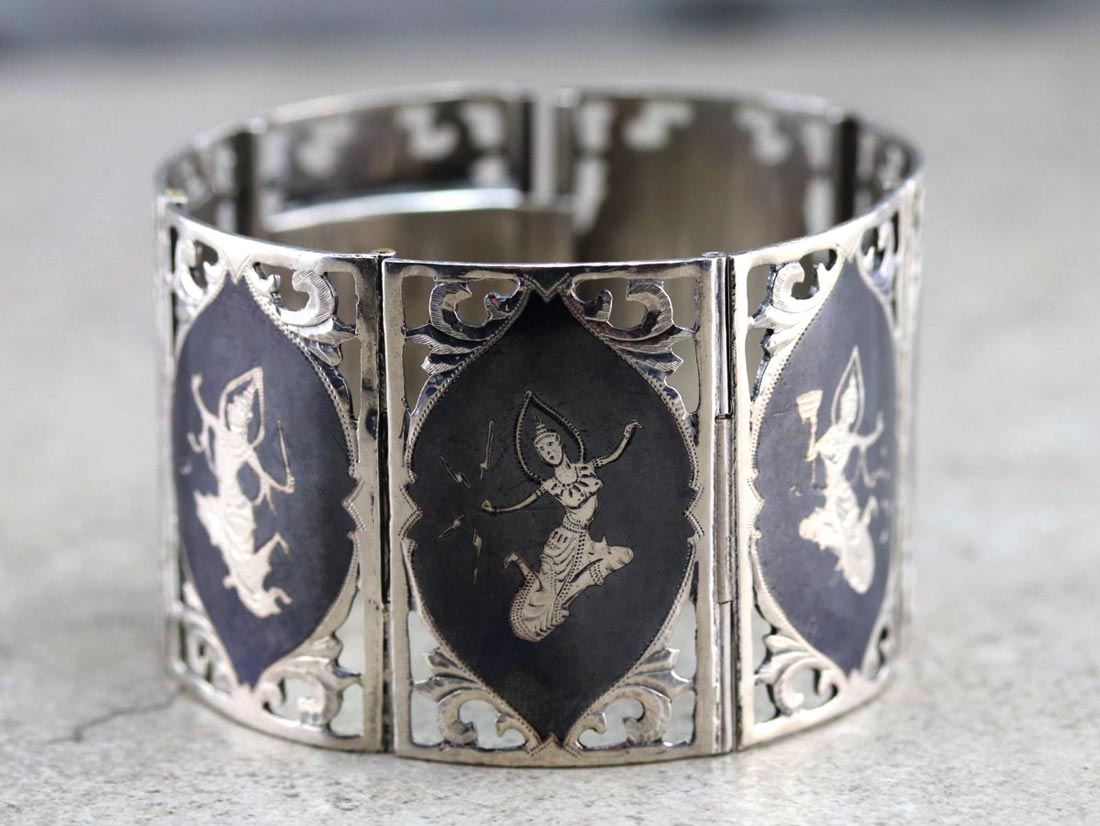The image depicts a gaudy piece of jewelry, either a bracelet or arm cuff, crafted from a silver or chrome-like metal. The item is placed upright on a marble table and comprises several hinged rectangular sections that come together to form a circular band. Each section is intricately designed with a regal appearance, featuring a detailed depiction of a woman. The woman, possibly inspired by ancient Egyptian or Hindu aesthetics, appears to be dancing in a semi-provocative manner while levitating items with her hands. She is dressed in skimpy, exotic clothing and wears a striking headdress. Some sections of the jewelry are in sharp focus, showcasing the woman's dynamic pose with arms extended and feet crossed, while others fade into the background, adding depth to the photograph.